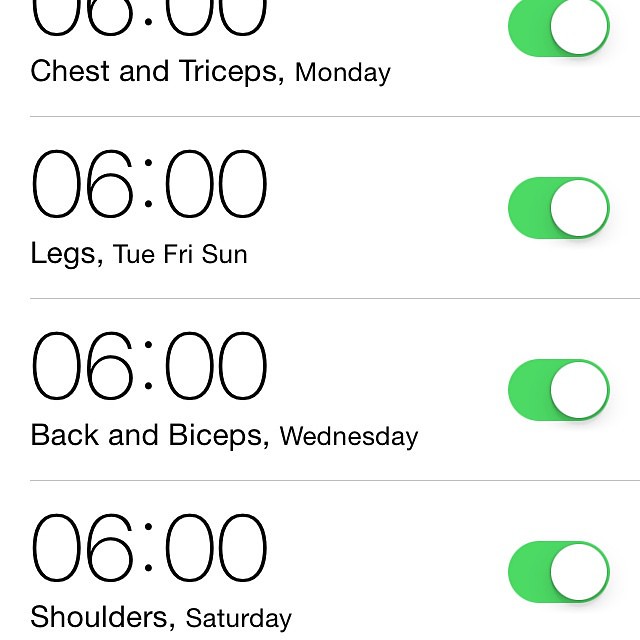The image is a screenshot from a smartphone displaying a workout schedule application. The screen has a white background with small lines that separate different sections, organizing the information clearly. There are four vertical sections on the right side of the screen with green toggle switches, each set to 'on' indicated by a white circle positioned to the right and a green highlight.

From top to bottom, each section lists a specific workout routine accompanied by the time and day. All workouts are scheduled for 06:00. The first section reads "Chest and Triceps Monday," the second notes "Legs Tuesday, Friday, Sunday," the third declares "Back and Biceps Wednesday," and the last states "Shoulders Saturday." The green toggles suggest that notifications for these routines are enabled.